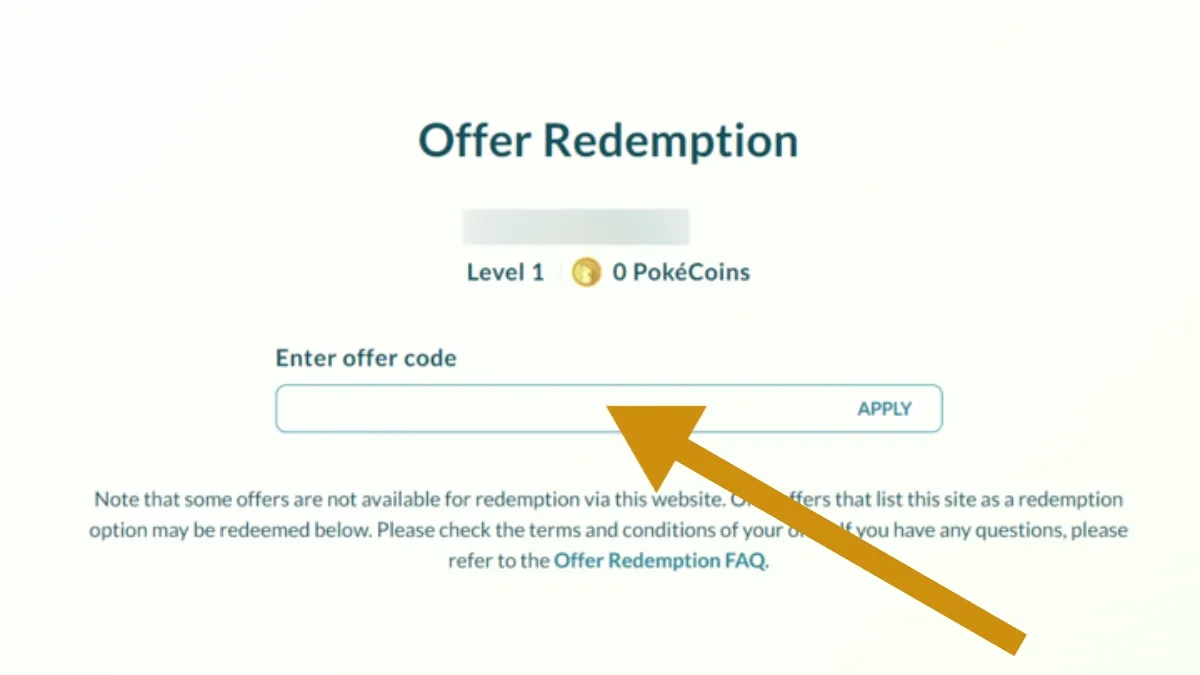The screenshot features a section of a Pokémon-themed website with a minimalist design on a white background. At the top, large bold letters in a shade of dark blue, nearly black, spell out "Offer Redemption." Below this heading, a rectangular box has been intentionally blurred out, likely concealing sensitive information such as a redemption code, a username, or a personal name.

Beneath the blurred section, the text "Level 1" is displayed, accompanied by an icon of a gold coin. The coin bears a white silhouette that closely resembles Pikachu. Next to this icon, the text specifies "0 PokéCoins," with the term "PokéCoins" clearly written, including the accented 'é' and a capital 'C.'

Further down, the instruction "Enter offer code" directs users to a long rectangular input box designed for entering the offer code. To the right of this box is a button labeled "Apply." Additionally, the screenshot is edited to include a large golden arrow pointing directly at the offer code input box, emphasizing its importance.